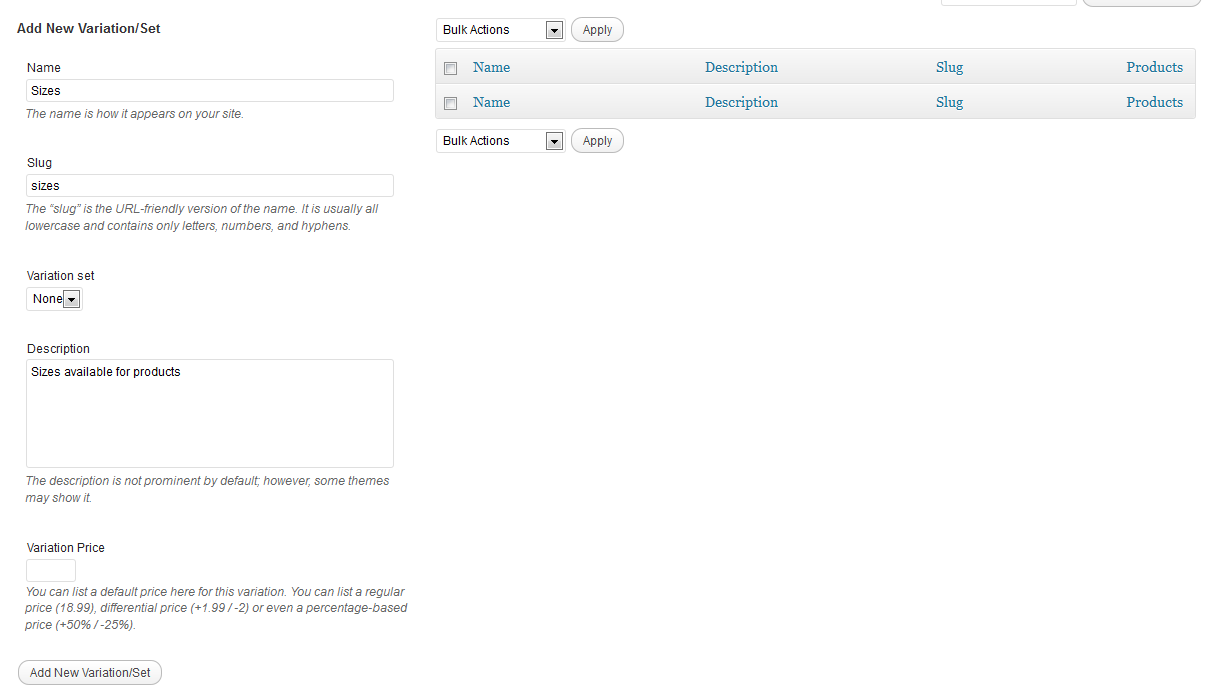In this image, we observe a detailed screenshot displaying a user interface for managing variations of a product on a website. The background is stark white, contrasted with black text for clarity. At the top, there is an instruction to "Add new variation set," indicating the feature to add different versions of a product.

Below, we see a structured box designed to input the product's name and available sizes. The "Name" field specifies how the product name will appear on the site, while the "Slug" field requires a URL-friendly version of the name, restricted to lowercase letters, numbers, and hyphens.

There is an area labeled "Variation set," which currently shows "None," and an expandable "Description" section, highlighting that while descriptions are not prominently displayed by default, certain themes may present them in bold text.

In the subsequent section, labeled "Sizes available for products," a white box is provided for entering the various sizes of the product. Moving down to the "Variation price" section, users can input default pricing information for the specified variation. Options include setting a regular price of $18.99, a differential price increase of $1.99, or even configuring a percentage-based price adjustment.

Towards the right side, the interface features a "Bulk actions" dropdown menu accompanied by an "Apply" action button, allowing multiple variations to be managed efficiently at once. The overall layout is clean and user-friendly, designed to facilitate the seamless management of product variations on an e-commerce platform.